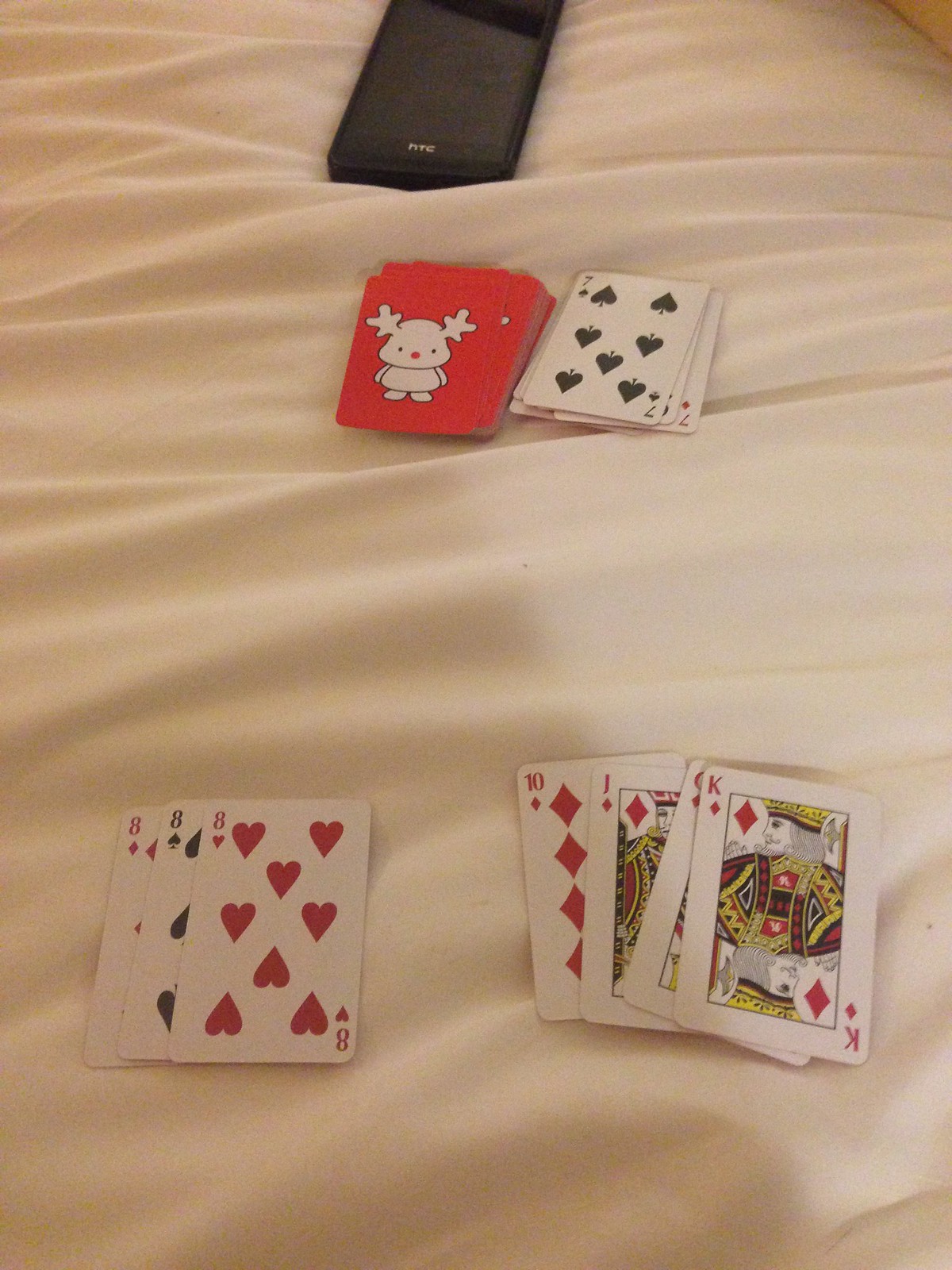The photograph depicts a bed with a white sheet that is noticeably wrinkled, suggesting someone recently laid across it. At the top center of the image, there is a black smartphone placed on the bed. Directly below the phone, still in the middle section of the frame, a stack of playing cards is visible. The top card on the stack features a reindeer with a red nose on a red background and is a seven of hearts. Arranged below the stack, three more cards are spread out: an eight of hearts, an eight of diamonds, and an eight of clubs, with the eight of clubs positioned in the center. To the right of these eights, there is a sequence of four cards: a ten of diamonds, a jack of diamonds, a queen of diamonds, and a king of diamonds, all sporting the distinct red suit. All these items rest atop what appears to be the bed mentioned earlier.